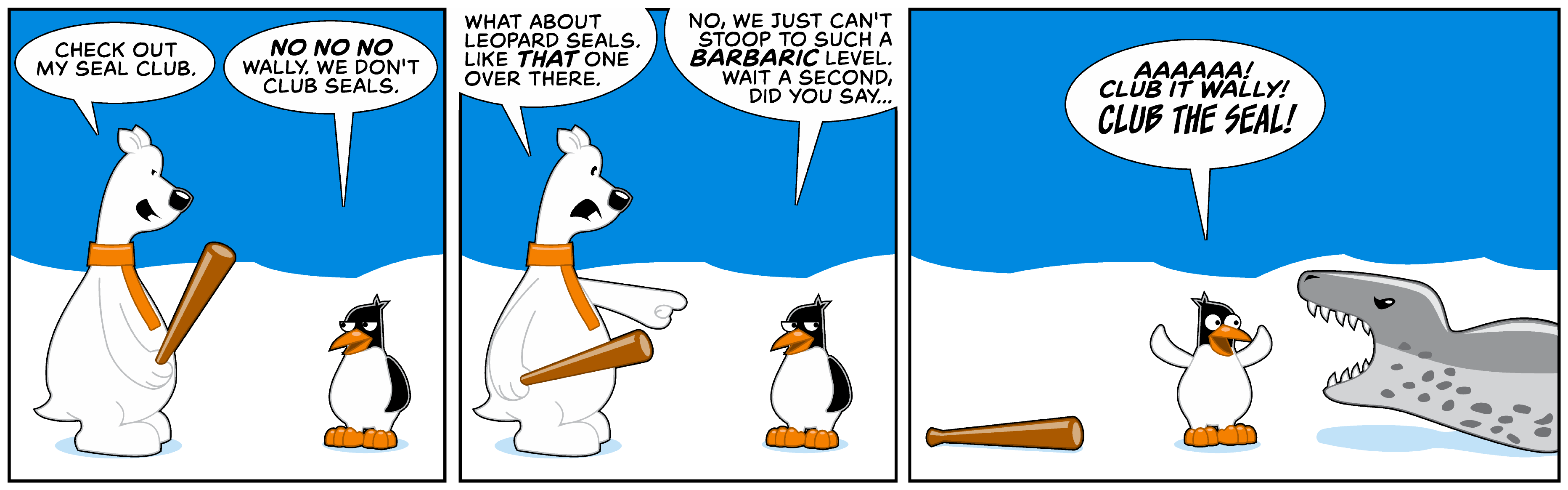The comic strip consists of three panels set in the Arctic, featuring a polar bear named Wally and a small penguin. Both characters are depicted standing on snow beneath a blue sky, and the polar bear is wearing an orange scarf. In the first panel, Wally, holding a club that resembles a baseball bat, proudly says, "Check out my seal club." The penguin, standing on the right, responds with concern: "No, no, no, Wally, we don't club seals." In the second panel, Wally points to a distance and asks, "What about leopard seals? Like that one over there?" The penguin replies, "No, we just can't stoop to such a barbaric level. Wait a second, did you say...?" In the final panel, the polar bear is gone, leaving the club on the ground, while the penguin, hands raised in panic, pleads, "Ah, club it, Wally, club the seal!" as a leopard seal with its mouth open and sharp teeth appears menacingly behind the penguin.